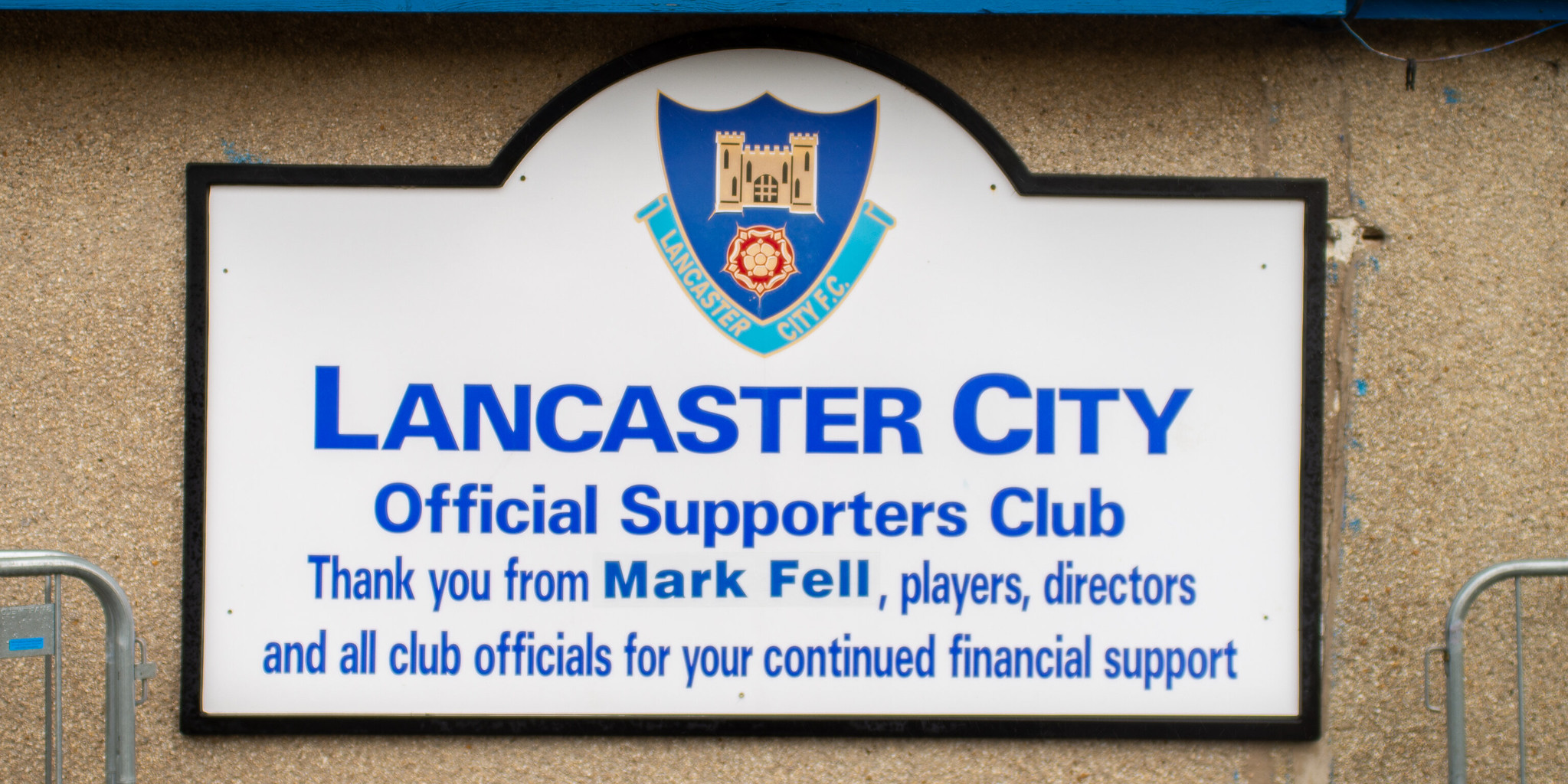This image captures a detailed scene of a plaque mounted on a rough textured, brownish stucco wall, suggestive of an outdoor location. Visible on either side of the plaque are the upper halves of bike racks, giving a sense of the area’s practical use. The plaque is rectangular with a beveled white surface trimmed in black, and it features an arched top. Prominently displayed at the top is a colorful emblem shaped like a shield, featuring a dark and light blue background, a small castle with two towers, and a reddish-gold flower below the towers. Inscribed in the light blue section of the emblem are the letters "Lancaster City F.C." Below the emblem, in bright blue letters, the plaque reads: "Lancaster City Official Supporters Club. Thank you from Mark Fell, players, directors, and all club officials for your continued financial support."